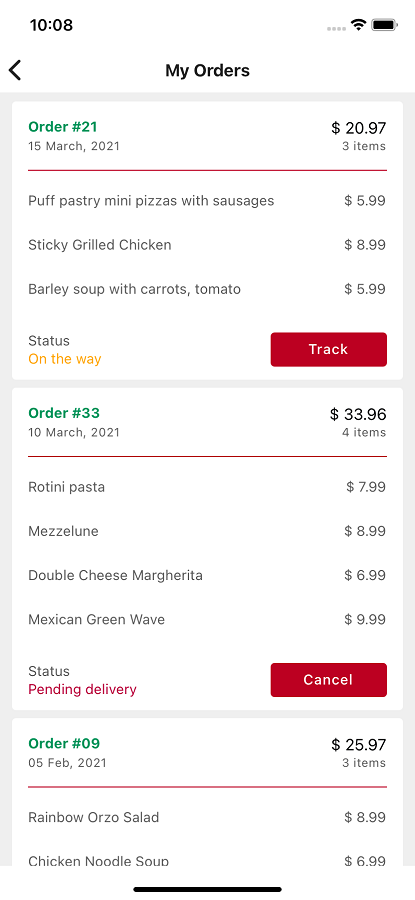This image is a detailed screenshot from an Apple phone, displaying a section of the user's order history within a food delivery app. The time shown on the phone is 10:08 AM, the battery is fully charged, and the Wi-Fi icon confirms an active internet connection.

At the top of the screen, there is a back button labeled 'My Orders'. Below it, the first entry is Order #21, placed on March 15th, 2021, totaling $20.97 for three items: Puff Pastry Mini Pieces with Sausage ($5.99), Sticky Grilled Chicken ($8.99), and Barley Soup with Carrots and Tomato ($5.99). The status of this order is marked as "On the Way", accompanied by a red 'Track' button.

The next entry is Order #33, made on March 10th, 2021, for a total of $33.96 consisting of four items: Rotini Pasta ($7.99), Mezze Lune ($8.99), Double Cheese Margherita Pizza ($6.99), and Mexican Green Wave ($9.99). The status of this order is "Pending Delivery" and features a red 'Cancel' button.

Lastly, there is an order placed on February 5th, 2021, for a total amount of $25.97. This order includes three items, though only two are visible: Rainbow Orzo Salad ($8.99) and Chicken Noodle Soup ($6.99).

Overall, the image effectively captures the detailed overview of several food orders, including their statuses and individual item details.